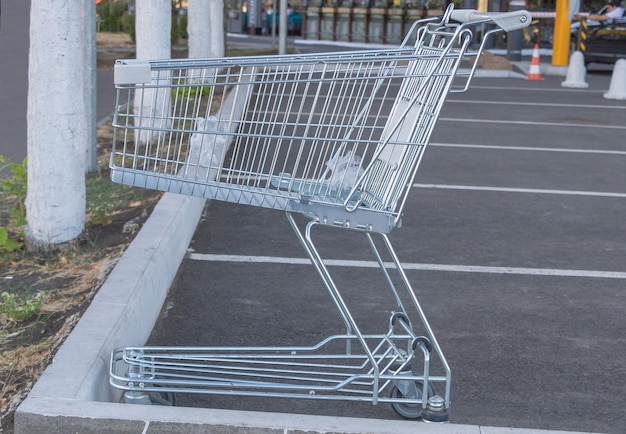In this all-too-familiar scene captured in a parking lot, an abandoned metallic steel grocery shopping cart with black wheels sits forlornly against a gray concrete curb. The parking lot's asphalt surface is neatly divided by white lines marking empty parking spaces. Beyond the curb, a small strip of land showcases patches of green grass, some brown dirt, and a few green-leafed plants. Concrete pillars rise from this median, standing like columns. The background reveals a blend of elements – yellow-painted posts, orange-and-white traffic cones, possibly some dirt, and indistinct windows. There is also a man visible in a vehicle, seemingly inserting a card into a gate, contributing to the bustle and slight disorder of the scene.